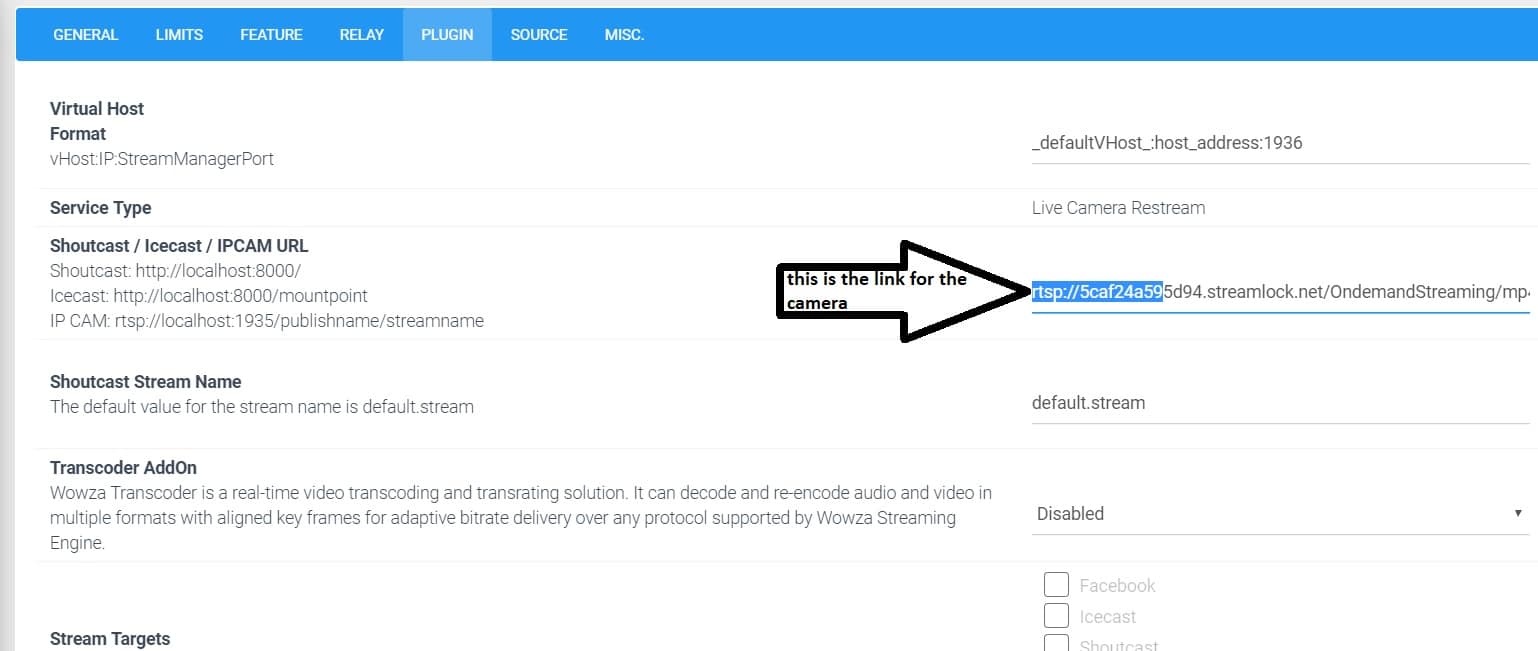The image is a horizontal screenshot of a webpage displaying a settings menu. At the top, there is a thin blue banner with a series of category tabs listed from left to right: General, Limits, Feature, Relay, Plugin, Source, and MISC. The "Plugin" tab is highlighted with a light blue box around it.

The left-hand side features a vertical column with specific settings options. Listed from top to bottom, these are: 

- "Virtual Host Format"
- "Service Type"
- "Shoutcast/Icecast/IPCam URL"
- "Shoutcast Stream Name"
- "Transcoder Add-on"
- "Stream Targets"

Further details are provided under these headings. On the right-hand side of the main page, beside "Virtual Host Format," there is an associated address. Under "Service Type," it specifies "Live Camera Restream." Adjacent to "Shoutcast/Icecast/IPCam URL" is a lengthy address, with the initial portion highlighted in blue. An outlined black arrow points to the start of this address, indicating it as the link for the camera.

Next to "Shoutcast Stream Name," it reads "Default.Stream." To the right of "Transcoder Add-on," a scroll-down button is labeled "Disabled." Below this, there are three unchecked boxes labeled "Facebook," "Icecast," and "Shoutcast," offering additional configuration options.